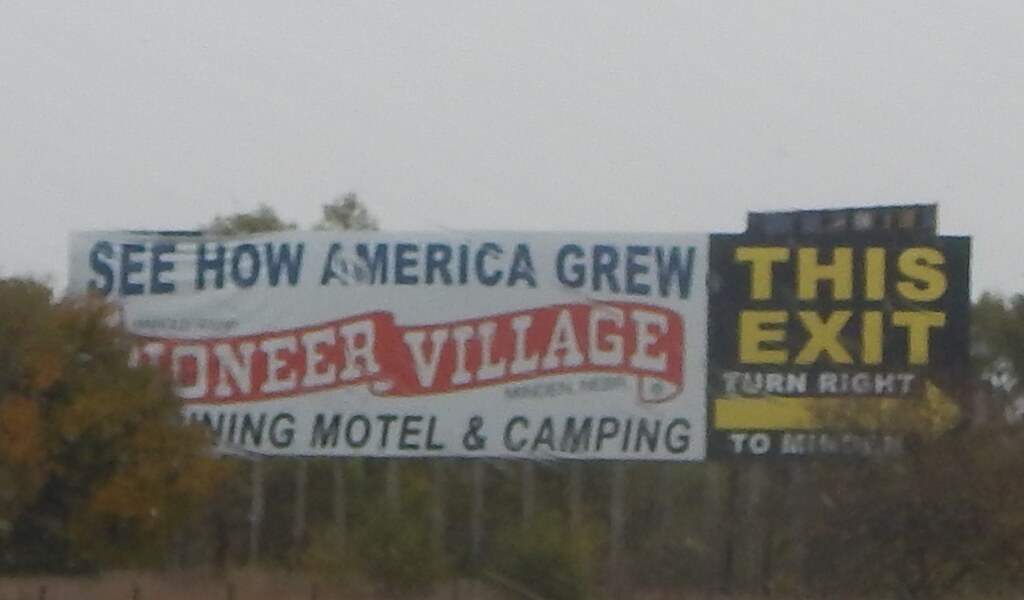A large billboard stands prominently amidst a cluster of green trees. On the left side of this billboard, there is a text that reads, "See How America Grew." Below this, partially obstructed by tree branches, a red banner displays the text "Pioneer Village." Further down, another partially hidden section suggests the phrases "Motel" and "Camping." To the right of the main billboard, a smaller black sign is attached, with an arrow and instructions that read, "This Exit Turn Right to [destination obscured]." Wooden poles support the billboard structure, and the entire scene is set against a backdrop of a gray, overcast sky.